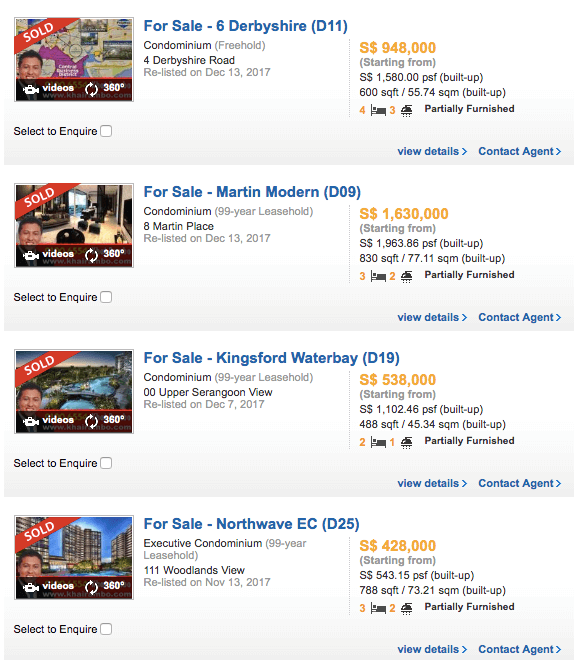Here is a refined and detailed caption for the given real estate website image:

---

The website showcases various real estate listings, predominantly featuring properties that have already been sold. 

1. The first listed property is a condominium located on Derbyshire Road. Initially offered for sale at $948,000, it has since been marked as sold. This freehold property, relisted on December 13, 2017, boasts a built-up area of 600 square feet (approximately 55.74 square meters) and includes four bedrooms and three bathrooms. It was partially furnished when listed. Contact details for the agent are provided, though the property is no longer available. 

2. The subsequent listing is also marked as sold, despite appearing under the "for sale" category. This condominium, named Martin Modern, features a 99-year leasehold and is situated at 8 Martin Place. Initially relisted on December 13, 2017, the asking price started at $1,630,000 but escalated to $1,900,000.

Overall, despite the 'for sale' tags, the properties displayed tend to be sold upon closer inspection, highlighting the high demand in the market.

---

This caption provides comprehensive details about the properties and clarifies their sold status while maintaining an organized structure.